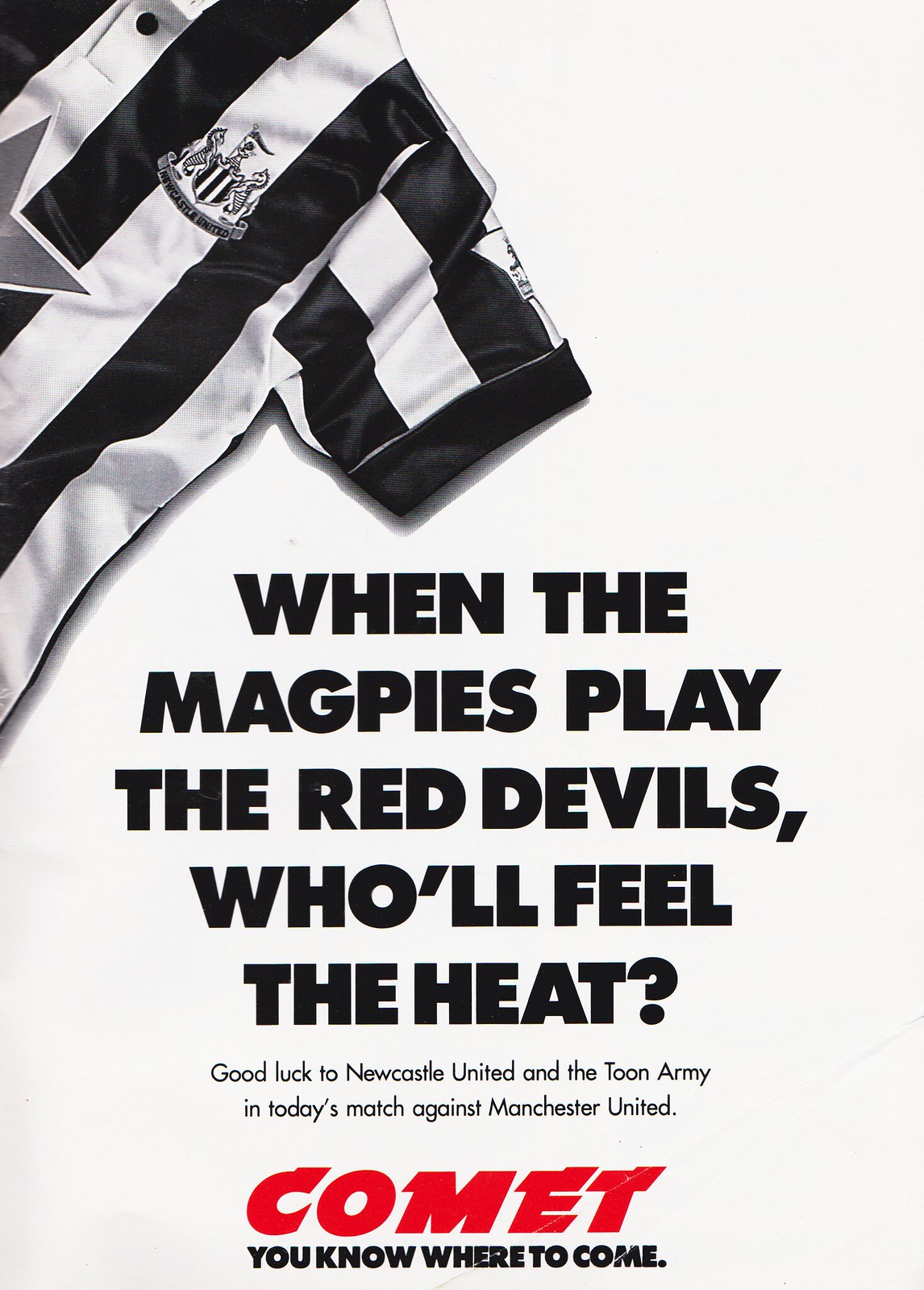The image resembles an advertisement poster on a faint light gray background, featuring the upper left portion of a black and white striped shirt, likely a Newcastle United uniform. The shirt’s torso displays thick vertical stripes, while the right sleeve has horizontal stripes, adorned with an emblem and a ribbon containing a coat of arms with horses, a flag at the top, and possibly a silver star. Dominating the center of the poster, bold black capital letters declare, "WHEN THE MAGPIES PLAY THE RED DEVILS, WHO WILL FEEL THE HEAT?" Beneath this, smaller black text conveys, "Good luck to Newcastle United and the Toon Army in today's match against Manchester United." At the bottom, "Comet" is emblazoned in large red letters, followed by the phrase "You know where to come" in black.